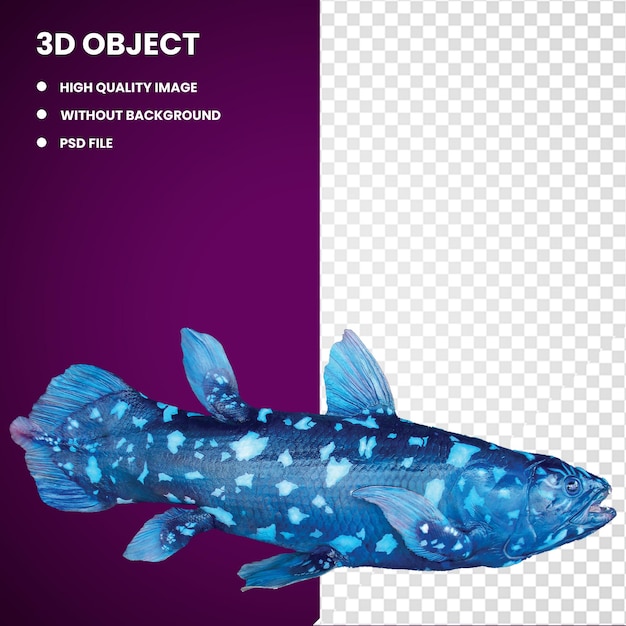The image showcases a high-quality 3D object displayed in a PSD file with no background. The backdrop is split into two sections: a dark purple segment on the left and a gray-and-white checkered pattern on the right. In the upper left-hand corner of the purple segment, white capital letters state “3D OBJECT” along with three bullet points that read: “high image quality,” “without background,” and “PSD file.” A striking 3D-rendered fish, possibly a fringe fish or an African coelacanth, is prominently featured spanning the purple and checkered segments. The fish is depicted in shades of blue with lighter blue spots, scales, and multiple fins. It has an open mouth, giving the impression of it swimming. The context suggests the image may be an advertisement for 3D modeling or printing services.